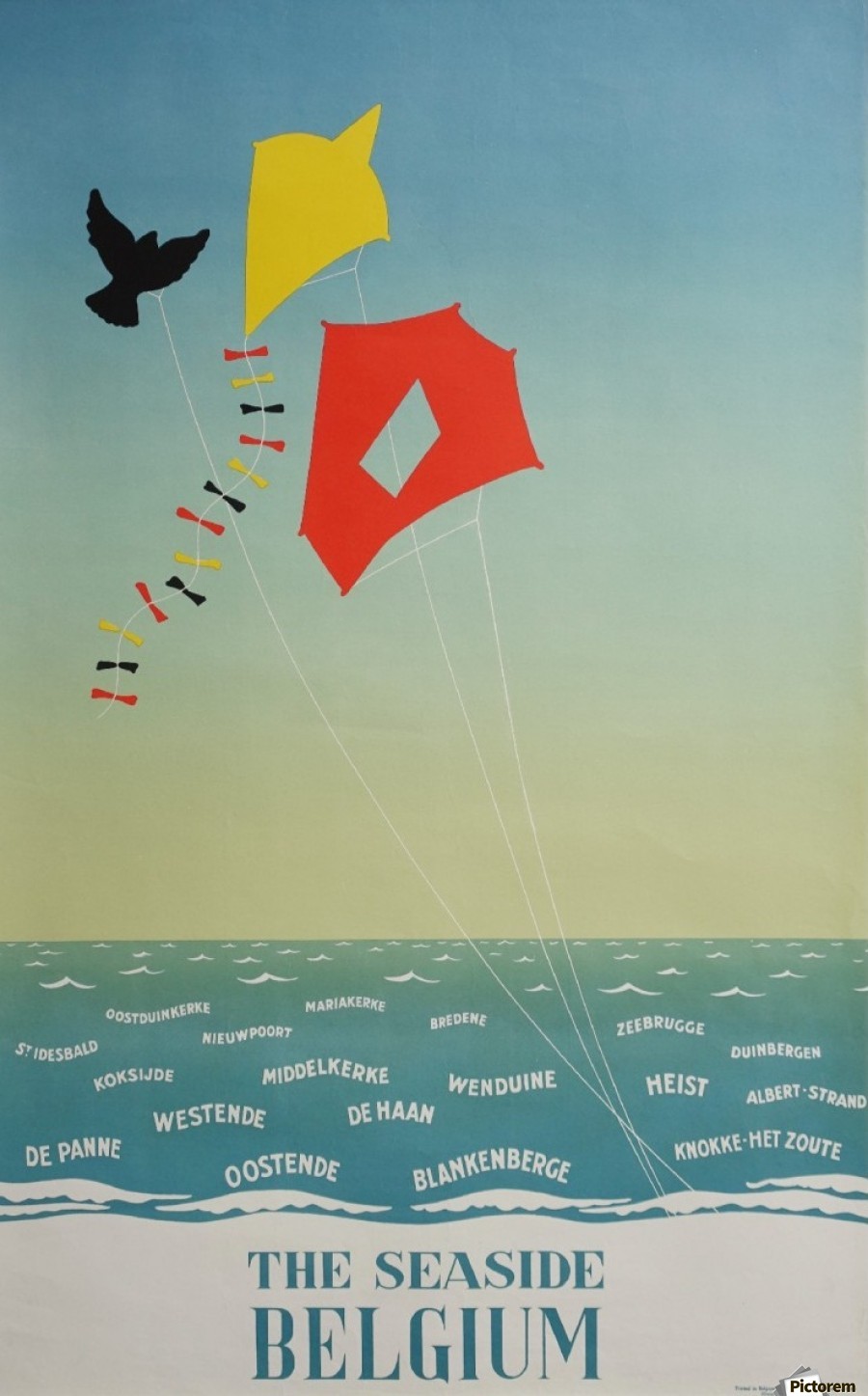The image is a vibrant advertisement for Seaside Belgium, depicted as an artistic rendering. The scenic illustration showcases a vivid, clear blue sky with the ocean stretched out beneath it, reflecting a serene and picturesque landscape. Three kites gracefully soar in the forefront, each distinct in design. A black kite shaped like a blackbird glides beside a yellow kite adorned with a tail of multicolored ribbons in red, yellow, and black. The third kite, striking in red, features a unique cutout in the center allowing glimpses of the sky to peek through. Each kite is tethered with a white string that extends down to a gray-hued ground. The waves of the sea are artistically inscribed with various words, possibly the names of Belgian coastal locations such as "Dipalm," "Winded," "Heist," which blend into the scene as part of the natural design. The bottom of the image prominently displays the tagline, "The Seaside Belgium," positioning the artwork as a captivating travel poster inviting one to explore the beauty and charm of Belgium's coastal regions.